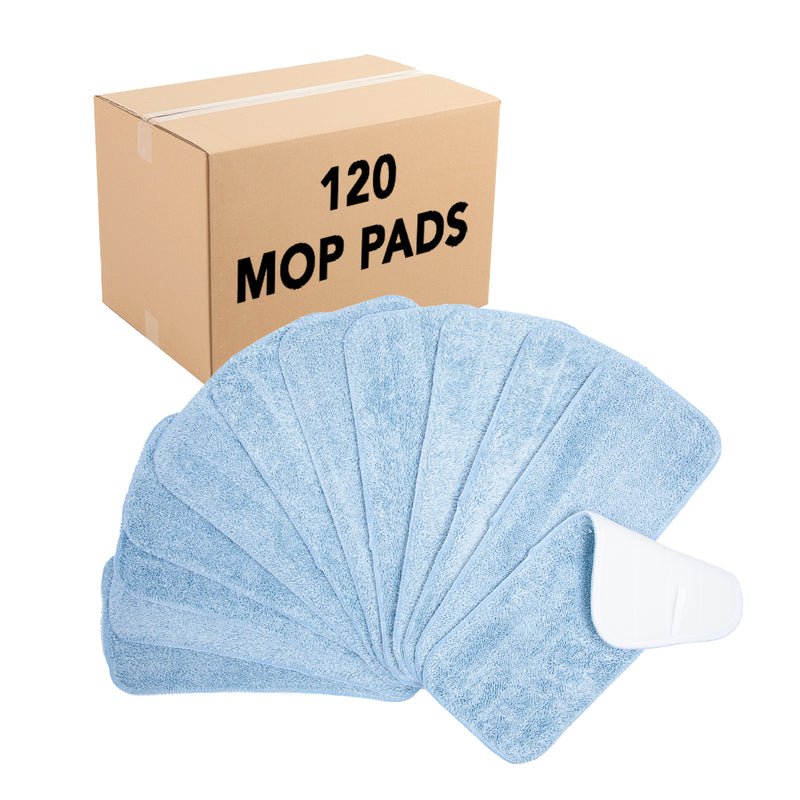In a stark white background, a slightly tilted brown cardboard box secured with white tape is placed in the upper left corner. The box, which measures around 18 by 18 or perhaps 24 by 18 inches, is plainly marked in black capital letters with "120 MOP PADS." Displayed prominently in front of the box are about 12 reusable mop pads, fanned out in a manner reminiscent of a clamshell. These mop pads are a pale, fluffy, light blue, made from terrycloth or microfiber material. Each pad is long, rectangular with rounded edges, and the furthest one on the right is flipped over, revealing its white backing, which may adhere to Swiffer-type mops. The overall display is simple and straightforward, focusing on clearly showcasing the mop pads.